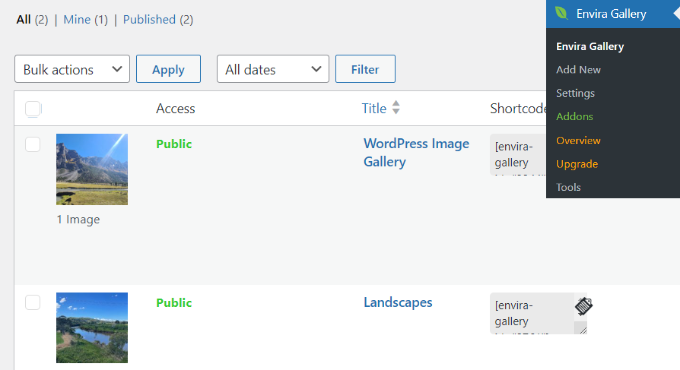Here's a detailed and cleaned-up caption for the given screenshot:

---

The screenshot captures a desktop application interface with a predominantly light gray background. In the top left corner, there are three clickable tabs— "All (2)," "Mine (1)," and "Published (2)"— with "Mine" and "Published" indicated in blue, suggesting they are hyperlinked.

In the top right corner, the page is branded with "Envera Gallery," accompanied by a green leaf logo on its left. Just below this branding, there is a navigation menu with the following options: "Add New," "Settings," "Add-ons," "Overview," "Upgrade," and "Tools." "Envera Gallery" is displayed in white font, "Add-ons" in green, "Overview" and "Upgrade" in orange, while "Add New," "Settings," and "Tools" are in gray.

The middle section of the screenshot features a tab labeled "Access," adjacent to which are columns labeled "Title" (with an up and down arrow for sorting) and "Shortcode." Under the "Access" tab, there are two entries for public photos. The first public photo showcases a nature scene with a mountain range and grassy terrain extending to the horizon. To its right, "WordPress Image Gallery" is written, and underneath it is the shortcode: "Envera-Gallery." The second public photo, directly below the first, depicts lush forests, a body of water in the middle, and a clear blue sky with several clouds. To the right of this photo, the title "Landscapes" is displayed, followed by the same shortcode: "Envera-Gallery."

---